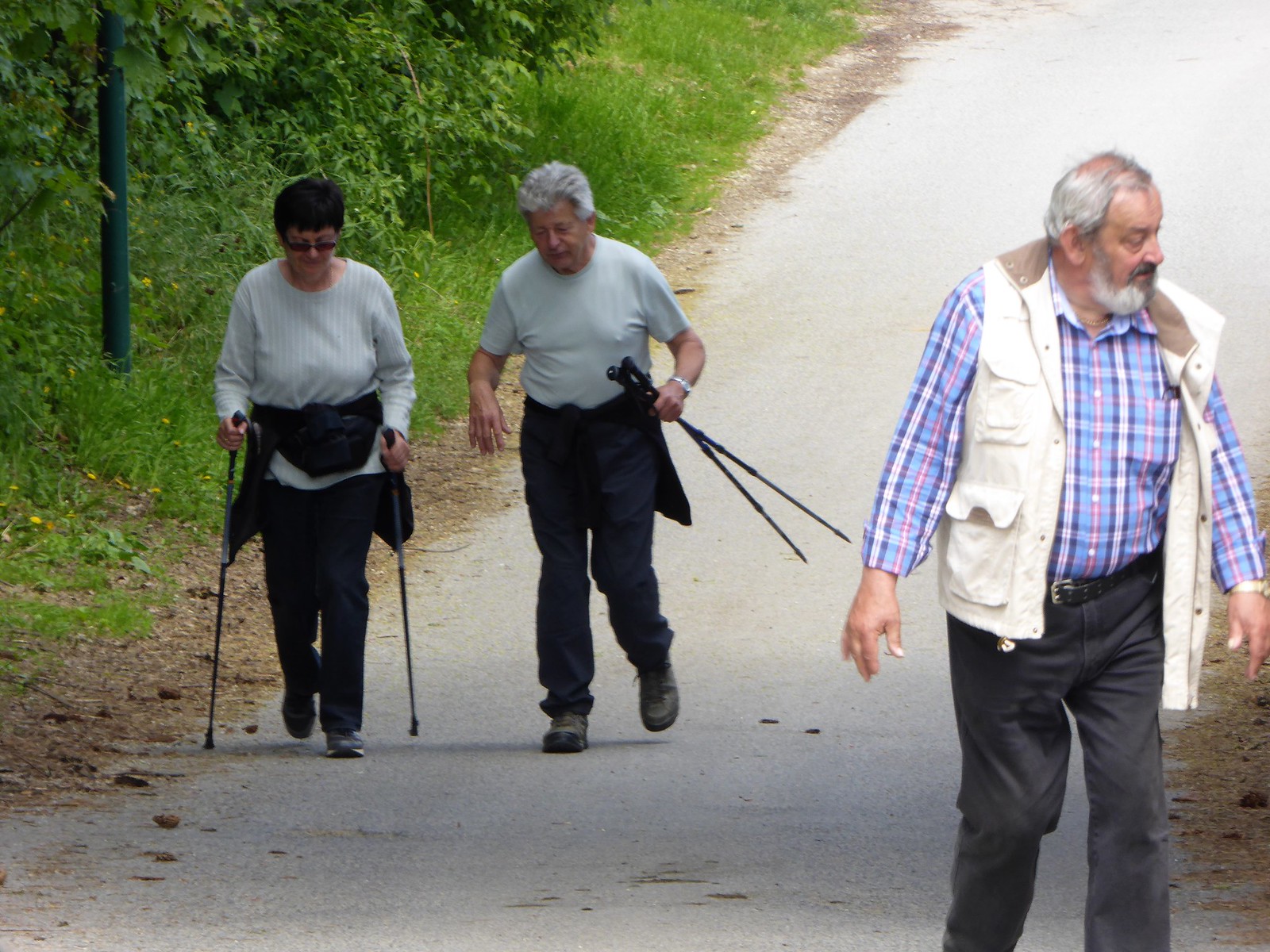This photograph captures three elderly individuals walking on a cement path lined with grass and dried pine needles. On the left side of the path, there is a lush mix of bushes, trees, and green grasses, punctuated by dandelion flowers. Leading the group is an older man wearing black jeans, dark shoes, a blue plaid long-sleeve shirt, and a cream-colored vest. He has a gray beard and is looking towards his right. Following him, walking side by side, are a man and a woman, both wearing black pants and gray shirts—the woman’s jacket is tied around her waist, and she uses walking poles in each hand, while the man carries his walking poles in his left hand and is also looking downward. The trio is immersed in a serene woodland setting, making their way along the winding path that disappears into the leafy distance.